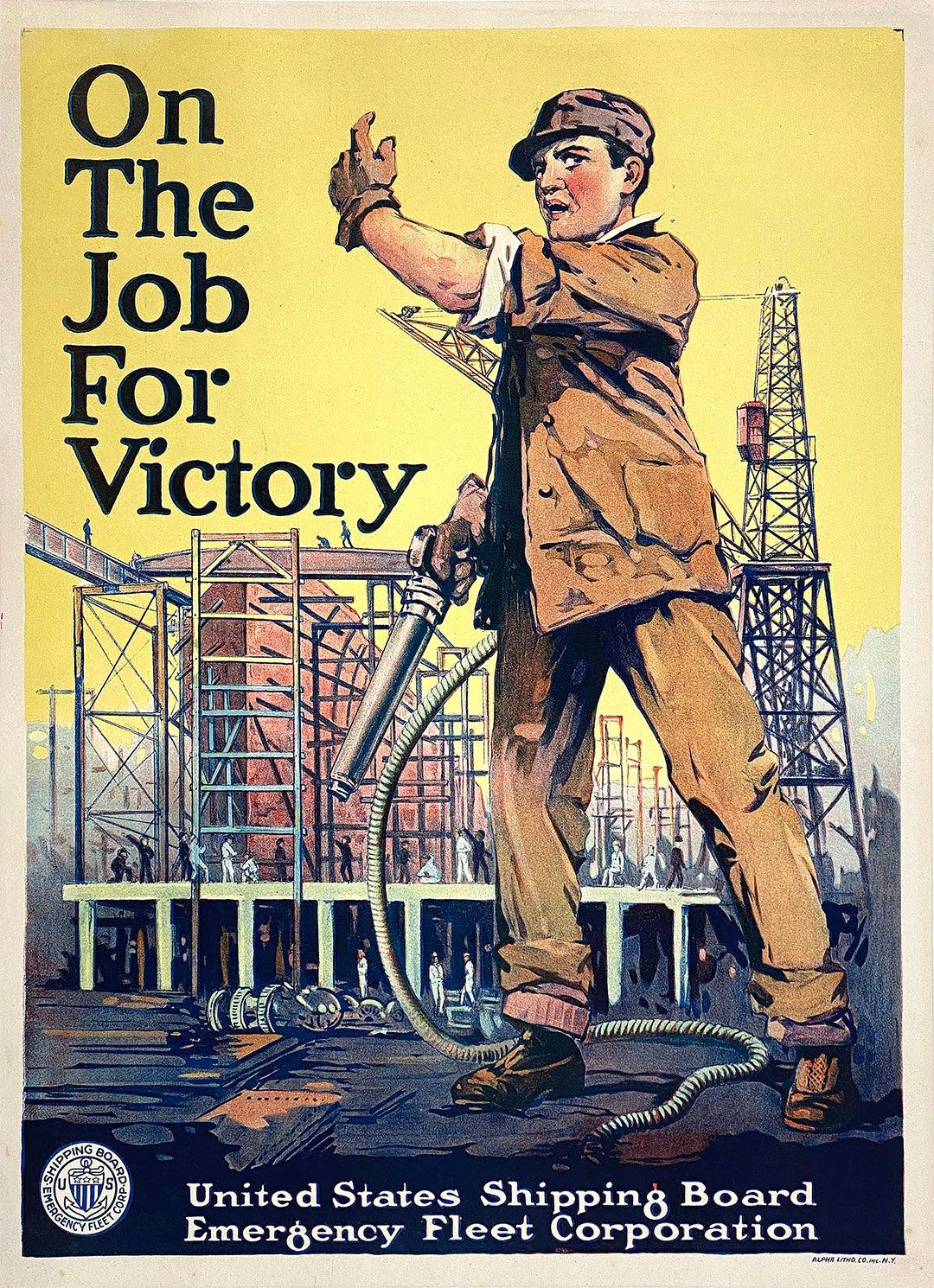This vintage poster, likely from the World War I or II era, prominently features the slogan "On the Job for Victory" at the top left corner and is branded with "United States Shipping Board, Emergency Fleet Corporation" at the bottom. The poster depicts a man at the center, dressed in a brown suit, brown trousers, brown shoes, a brown hat, and brown gloves. The man, possibly Caucasian with light-colored skin, appears to be holding a gray or silver welding tool with a long hose. He stands in front of an industrial backdrop featuring an old crane and several workers. His expression conveys fear or alarm. The background is a striking yellow, enhancing the sense of urgency and wartime effort conveyed by the poster. The bottom left corner includes the logo of the United States Shipping Board Emergency Fleet Corporation, written in blue.